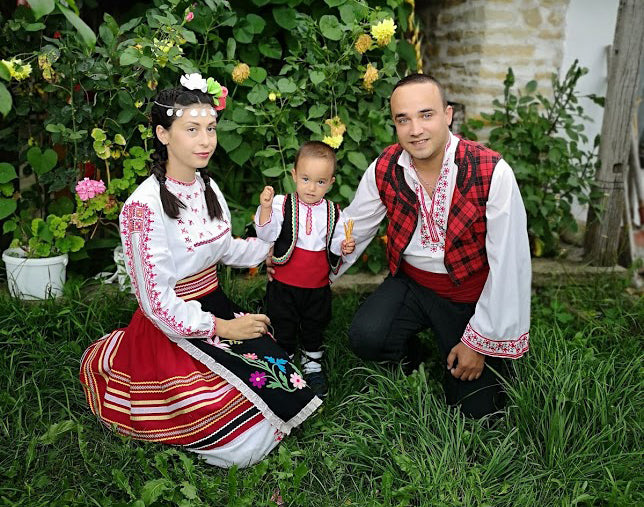This detailed photograph captures a family of three dressed in traditional, elaborate outfits posing in an outdoor setting. The woman on the left has her dark hair styled in pigtails adorned with flowers and a headdress. She is wearing a white blouse with red checkered detailing down the sides, an apron, and a white dress featuring a colorful red skirt with yellow pleats. The man on the right is dressed in a long flowing white shirt with similar red embroidery on the sleeves, paired with a plaid vest, black pants, and a thick, red belt sash. The young boy standing between them, about two or three years old, mirrors his father's attire with a black vest, white shirt with red detailing, black pants, and a red sash, creating a cohesive family appearance. They are all kneeling, except the child, who stands on a patch of wild, unmanicured grass. Surrounding them is a verdant scene with tall grass, green bushes, pink geraniums, yellow flowers—possibly roses—and a stone wall in the background to the right. This image, rich with cultural authenticity, doesn't specify the country of origin but indicates they are not dressed in American attire.